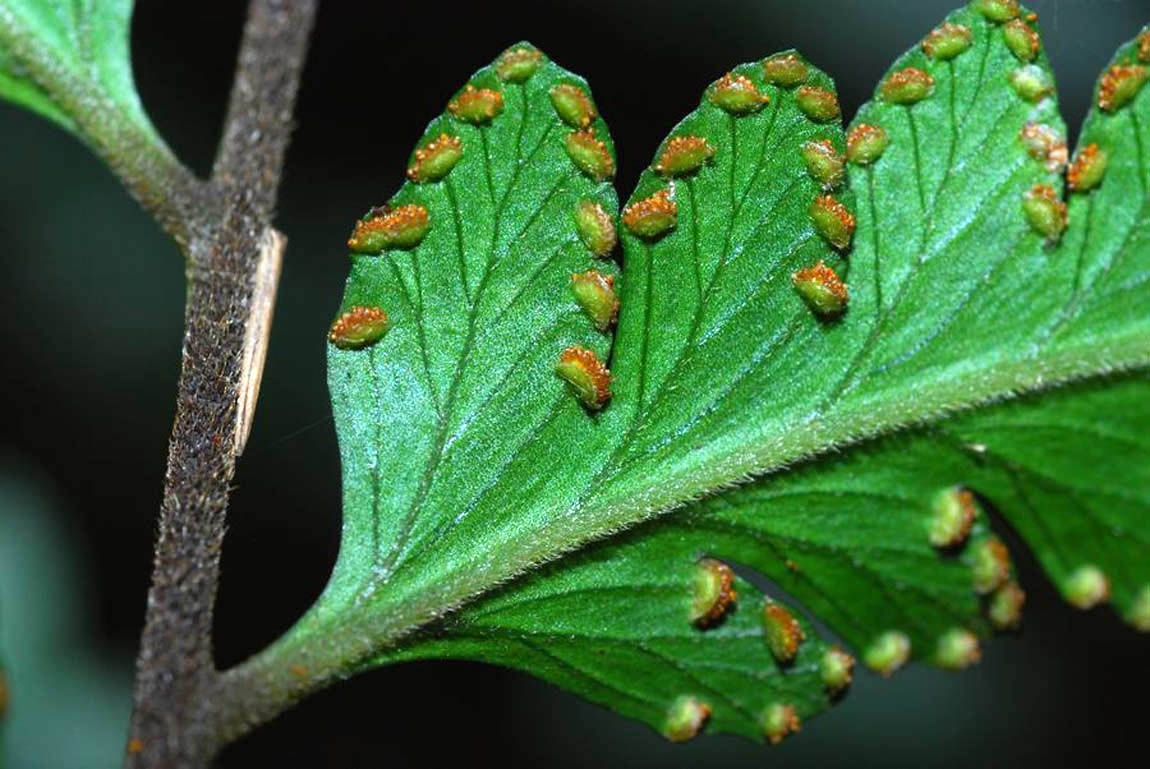The close-up photograph depicts the underside of a green, possibly non-tree leaf that appears to be part of a compound structure, featuring multiple leaflets branching from a thin, almost fragile-looking stem. The leaf has a fuzzy, almost furry texture, particularly along its central vein, with a deepening green color as it extends outward from the center. Notably, the underside of the leaf is covered with an array of small, green taco-shaped structures outlining every segment of the leaf. These structures, which could be insect eggs or larvae, have a green base sprinkled with a cream-colored substance resembling cheese. These egg masses or seed-like forms suggest a common insect-laying behavior on the plant. The main stem from which these leaves extend has a grayish or brownish tint, adding to the contrast. The entire image is captured outdoors, highlighting the unique characteristics of this intriguing leaf.